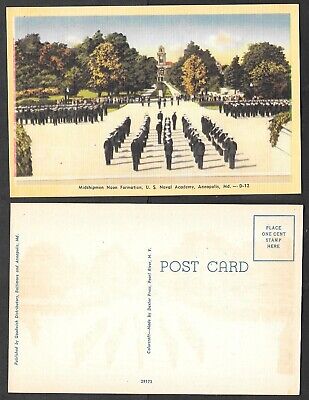The postcard features a vintage photograph of the U.S. Naval Academy midshipmen in formation. The scene captures numerous soldiers clad in white hats and black or dark navy blue uniforms. They are neatly aligned in rows across a large courtyard or square, with distinct groups positioned to the left, right, and center. The backdrop of the image is a tall building with a prominent tower, encircled by lush, tall trees. The angle of the shadows indicates that it is daytime with the sun lower in the sky. The postcard itself has a white bottom section labeled "Postcard," and a designated area in the top right corner for a one-cent stamp. The framing around the image is cream-colored, and there is some text beneath the photograph, though it's too small to read clearly.